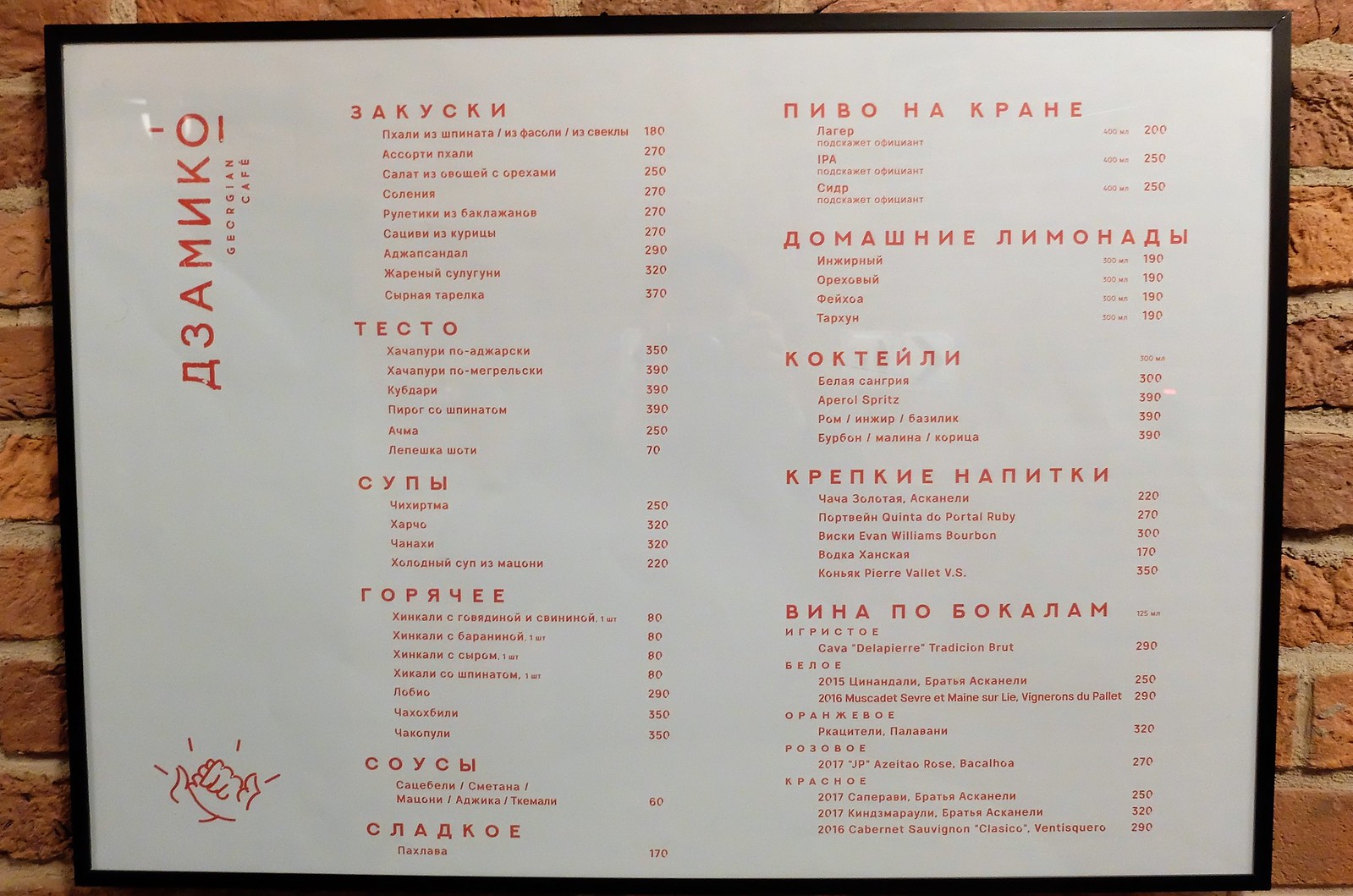A detailed caption for the image could be:

"A framed restaurant menu hung on a brick wall with a sleek black frame. The menu, written entirely in red lettering in a foreign language, features an extensive list of options organized under distinct headers and subcategories, with prices aligned to the right. The restaurant's name, also in red lettering, is situated in the upper left-hand corner, though it is oriented sideways, making it difficult to read. The lower left corner of the menu displays an illustration of two clasped hands, encircled by radiating red lines. The text is very small, and there are no pictures of food, making it challenging to decipher any specific details."